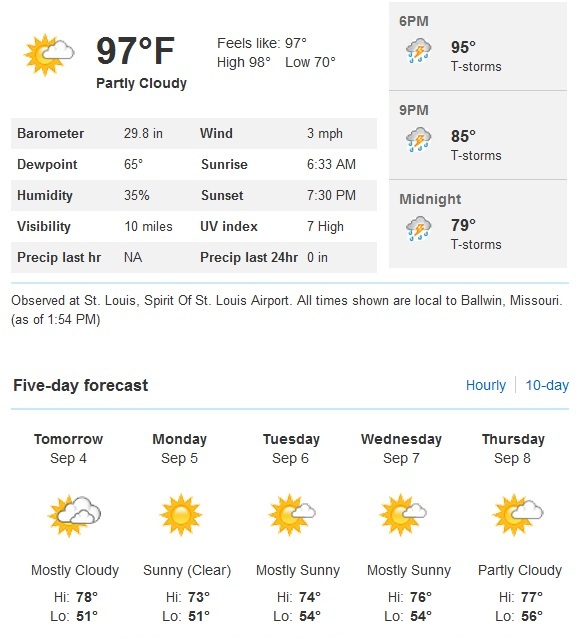**Weather Report for Baldwin, Missouri Observed at Spirit of St. Louis Airport as of 1:45 PM**

- **Current Conditions:**
  - **Temperature:** 97°F (Feels like 97°F)
  - **Weather:** Partially Cloudy
  - **High:** 98°F
  - **Low:** 70°F
  - **Barometer:** 28.6 in
  - **Dewpoint:** 65°F
  - **Humidity:** 35%
  - **Visibility:** 10 miles
  - **Perception:** 0 inches in the last hour, and last 24 hours
  - **Wind:** 3 mph
  - **UV Index:** 7 (High)
  - **Sunrise:** 6:33 AM 
  - **Sunset:** 7:30 PM 

- **Weather Forecast:**
  - **6 PM:** 95°F, Thunderstorms (icon: cloud with lightning and rain)
  - **9 PM:** 85°F, Thunderstorms (icon: cloud with lightning and rain)
  - **Midnight:** 79°F, Thunderstorms (icon: cloud with lightning and rain)

- **Upcoming Days:**
  - **Tomorrow, September 4:** Mostly Cloudy, High 78°F, Low 51°F
  - **Monday, September 5:** Sunny and Clear, High 75°F, Low 51°F
  - **Tuesday, September 6:** Mostly Sunny, High 74°F, Low 54°F

*All times shown are local to Baldwin, Missouri.*